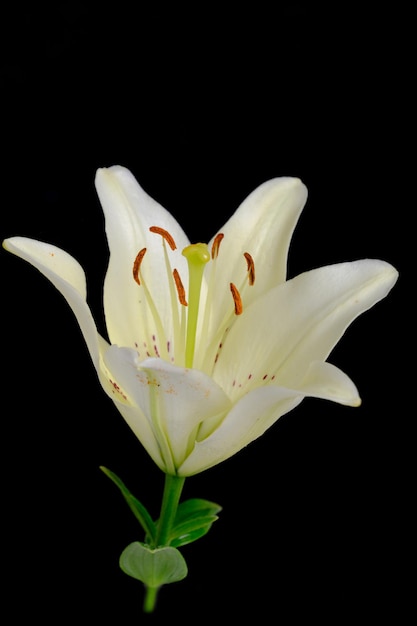The image showcases a single white lily in full bloom, positioned centrally against a completely black background. The lily's five to six pristine white petals, each detailed with fine linings and slight spotting near the base, are elegantly opened, revealing the intricate structure of its inner organs. At the heart of the flower, six slender green stamens topped with vibrant yellow-orange pollen surround the central green stem. This green stem is adorned with three leaves, adding a touch of natural greenery. The entire flower is bathed in even, well-balanced lighting, emphasizing its photorealistic botanical beauty without any visible shadows. The background and foreground remain entirely devoid of any distractions, ensuring the lily is the sole, striking focus of the image.